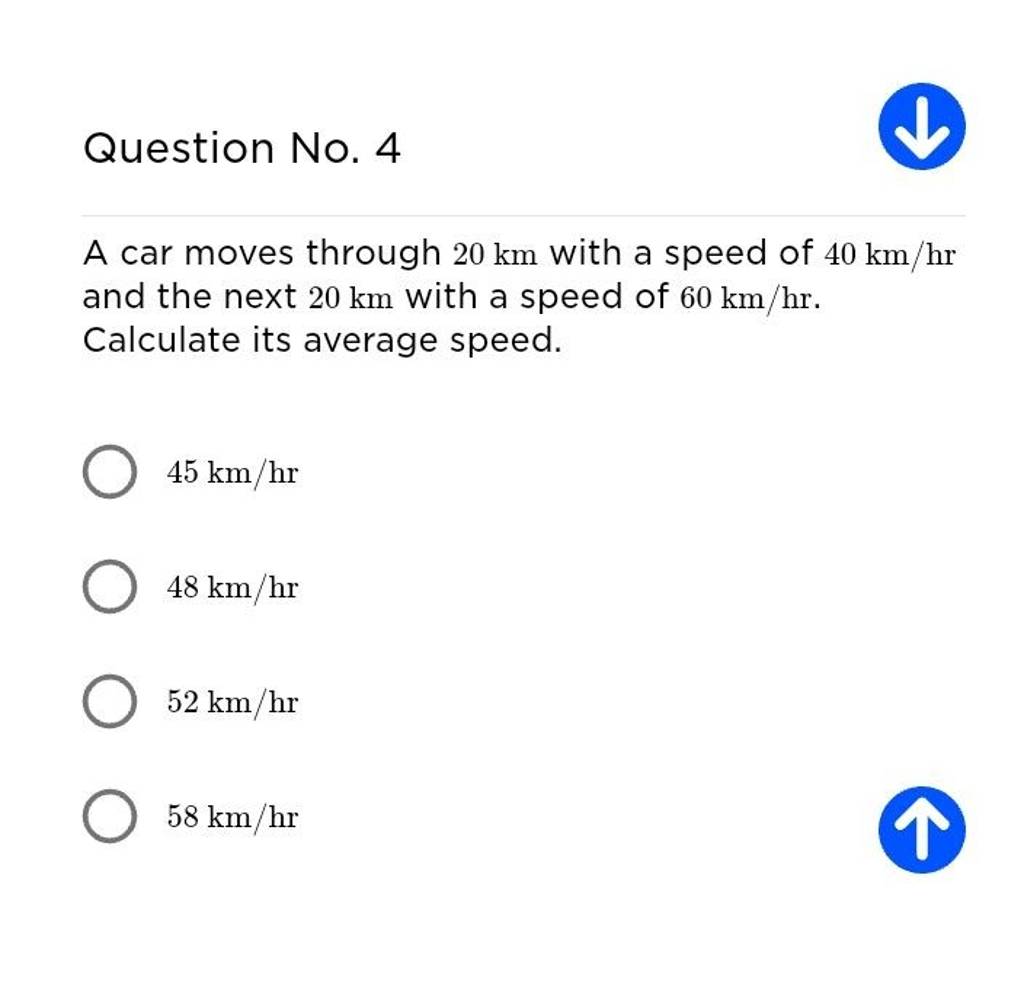This screenshot features a quiz question labeled "Question No. 4" at the top, written in larger font. On the right side, a blue circle with a white downward arrow is visible. The question itself reads: "A car moves through 20 km with a speed of 40 km/hr and the next 20 km with a speed of 60 km/hr. Calculate its average speed." Immediately below the question are four options, each accompanied by a clickable gray circle with a white center: 

1. 45 km/hr
2. 48 km/hr
3. 52 km/hr
4. 58 km/hr

Additionally, at the bottom right of the image, there is another blue circle with a white upward arrow, suggesting navigation. The measurements for speed are denoted as "km/hr." This detailed depiction highlights the structure and elements of the quiz question interface.